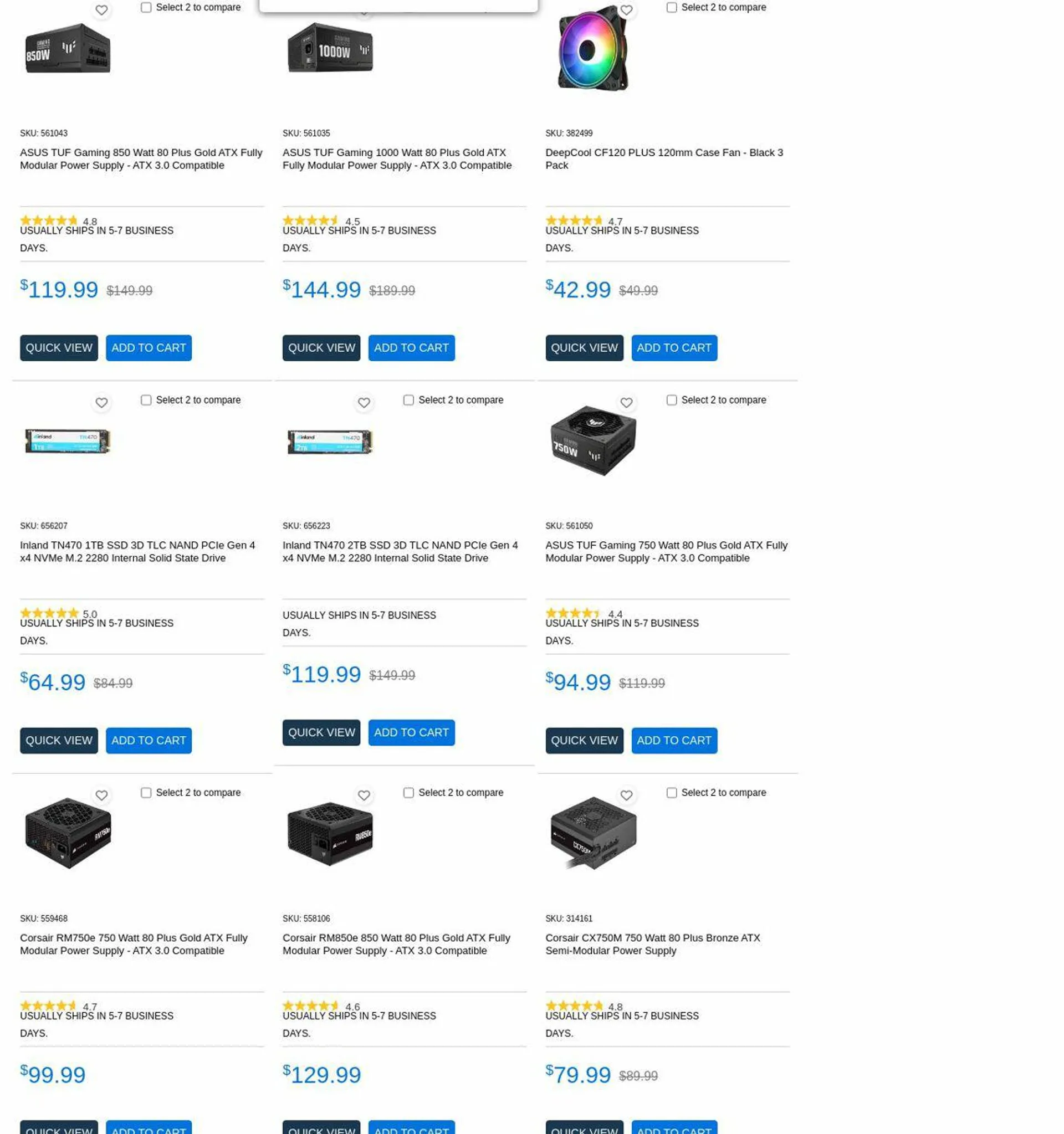A person is shown holding a smartphone, engaged in an online search for gaming accessories. On the screen, nine products are displayed in a grid format, organized into three rows of three items each. Each product appears within a card-like area, providing comprehensive information without any borders. These details include a product image, SKU number, customer rating in stars, a brief description, estimated shipping time, the current price, the original price (if discounted), and two buttons for 'Quick View' and 'Add to Cart.'

In the top row:

1. Two identical "Gaming Plus Gold Power Supplies."
2. A three-pack of case fans.

In the middle row:

1. An internal solid state drive (SSD).
2. Another internal solid state drive (SSD) at a different price.
3. A power supply.

In the bottom row:

1. Another power supply.
2. Another identical power supply.
3. Yet another power supply.

The screen offers a mixture of gaming power supplies, cooling systems, and storage devices, all essential components for building or upgrading a gaming PC.